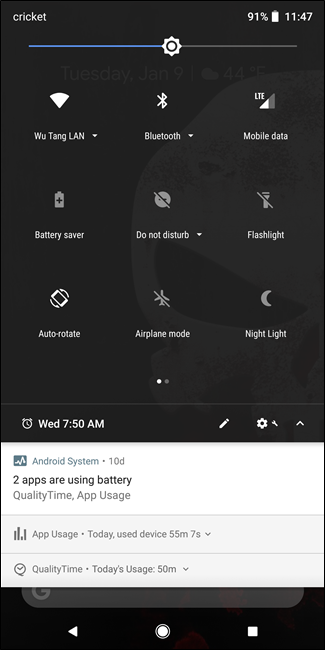Screenshot of a Smartphone Display:

The screenshot showcases a smartphone display. At the top left corner, the word "Cricket" appears in white letters, indicating the carrier. On the top right, the battery status shows "91%" with a full battery icon next to it, and the time reads "11:47."

Below this, there is a progress bar, about halfway filled, with a gear icon in the center, suggesting a loading or configuration process. The bar is blue in the filled portion and gray in the unfilled.

Under the progress bar, there are several icons, each with a downward arrow indicating more options. These icons represent:

- Wi-Fi, denoted by a symbol and the text "WU-TANG-TANG-LANG."
- Bluetooth, indicated by the Bluetooth icon next to the word "Bluetooth."
- Mobile data, shown with a series of bars and the text "LTE."

Three more icons are listed below:

- Battery Saver, represented by a battery icon with a black plus sign inside it.
- Do Not Disturb, shown with a circle and a diagonal line through it.
- Flashlight, depicted with a flashlight icon and a diagonal line crossing from upper left to lower right.

Further down, three additional icons are present:

- Auto-Rotate, depicted with a phone icon indicating rotation.
- Airplane Mode, shown with an airplane icon and a diagonal line.
- Night Light, illustrated by a crescent moon icon.

A gray bar separates the following section, which contains a small white clock, the day ("WED"), and the time "7:50 a.m." To the right are icons for editing and settings, including a white pencil, a gear, a wrench, and an upward triangle.

Below this section, an area displays "Android System" with a blue square and a white squiggly line next to it. A small black text reads "10d," and beneath it, "2 apps are using battery." Another gray bar leads to detailed app usage statistics, listing:

- "Quality Time, app usage," along with a total usage figure.
- A detailed breakdown showing "Today, used device 55 minutes 7 seconds" with a downward arrow.
- Another entry for "Quality Time" with "Today's usage 15 minutes" and a downward arrow.

At the bottom of the screen, a rounded rectangular search bar with the letter "G" (representing Google) is centered. On either side of this bar, there are navigation icons: a back arrow on the left, a home circle in the center, and a square for recent apps on the right.